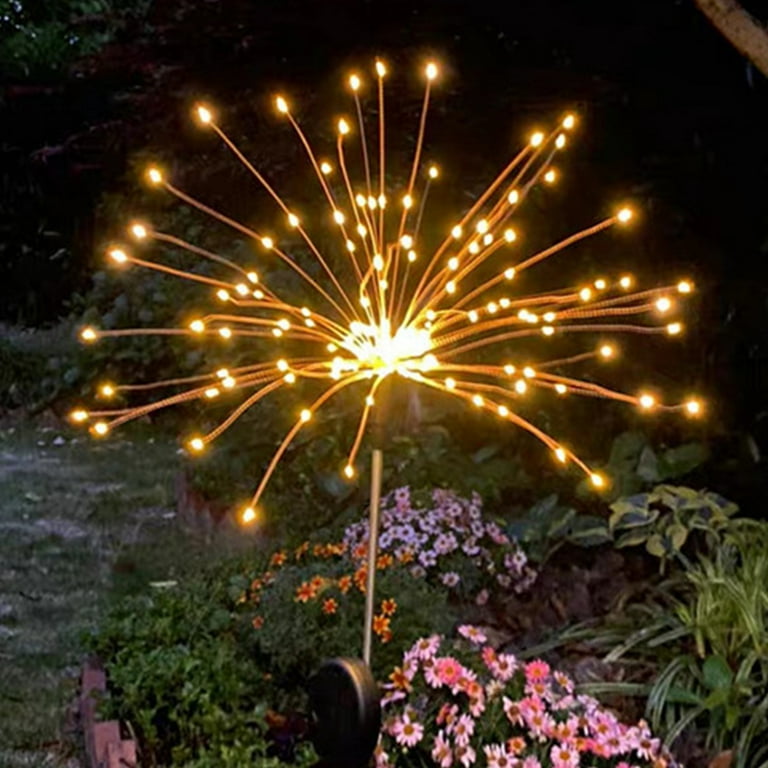In a serene nighttime garden, a striking sculpture stands illuminated against a dark backdrop. This contemporary piece, resembling a gigantic dandelion made from copper wire and LED lights, captures the eye with its intricate design. The sculpture features numerous strands radiating from a brilliantly lit center, each ending in a bright light, with some intermediate lights along the strands. These radiating wires, resembling sparkler trails, give the illusion of a dandelion dispersing its seeds into the night. The structure is supported by a metal pole anchored firmly in a flower bed adorned with vibrant vegetation. Below the sculpture, an array of pink, purple, and orange flowers in various shades of green fill the plant bed, bordered by decorative brick edging. The surrounding garden is lush with a variety of plants and trees, enhancing the magical ambiance of this illuminated spectacle.